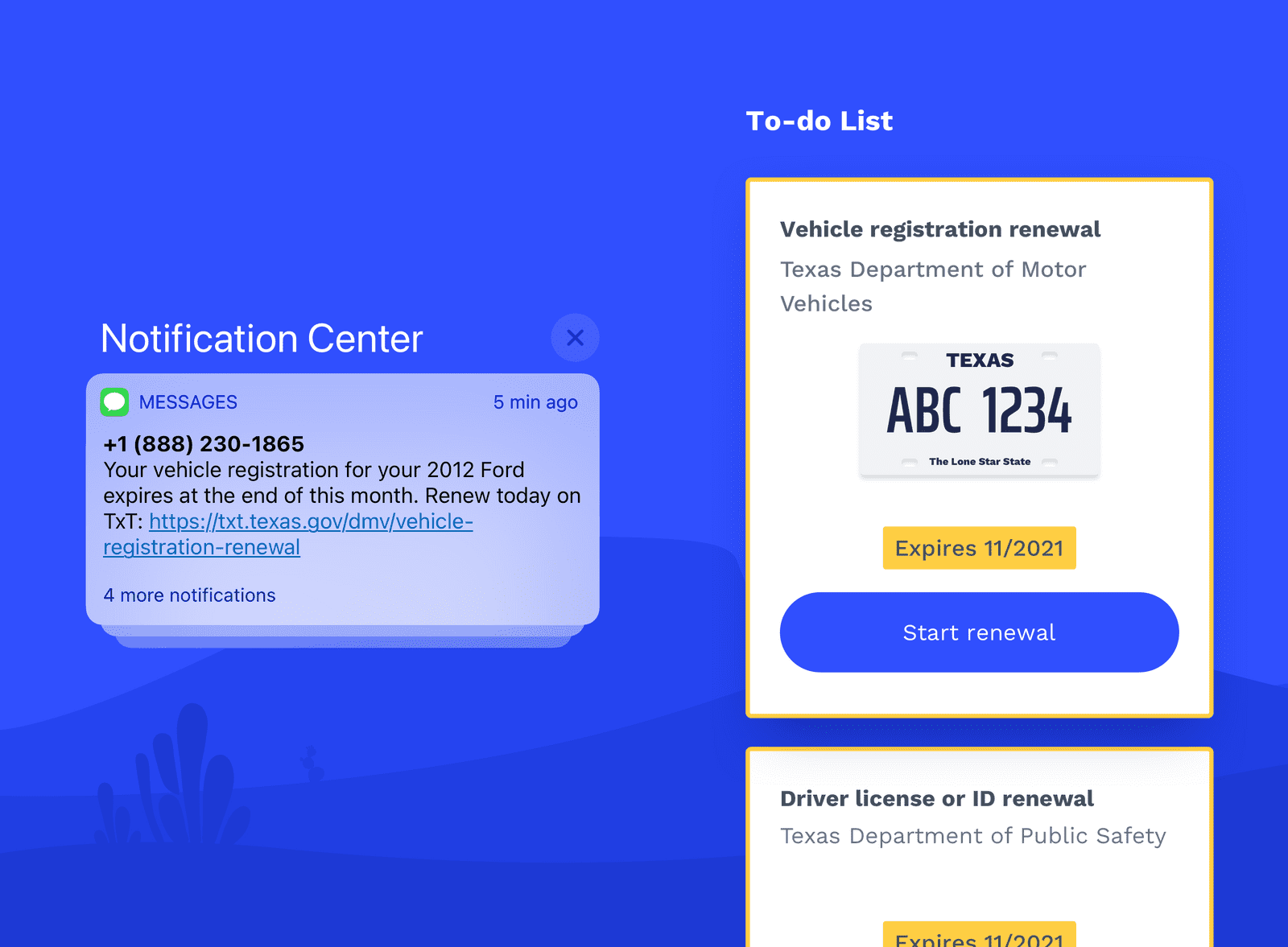A vibrant landing page for the Texas Department of Motor Vehicles (Texas DMV) focused on vehicle registration renewal. The header features the text "To-Do List" against a bright blue background. The lower section showcases stylized artistic layers of blue, forming abstract dunes, hills, and a cactus. On the left-hand side, a notification center displays important messages, including a prominent alert that your vehicle registration for your 2012 Ford expires at the end of this month, accompanied by a link for immediate renewal. Four additional notifications are listed under this. On the right side, there is an area dedicated to "Vehicle Registration Renewal", adorned with an image of a Texas license plate that prominently displays an expiration date of "11 2021" in yellow. A striking blue button with white text labeled "Start Renewal" invites users to begin the renewal process.